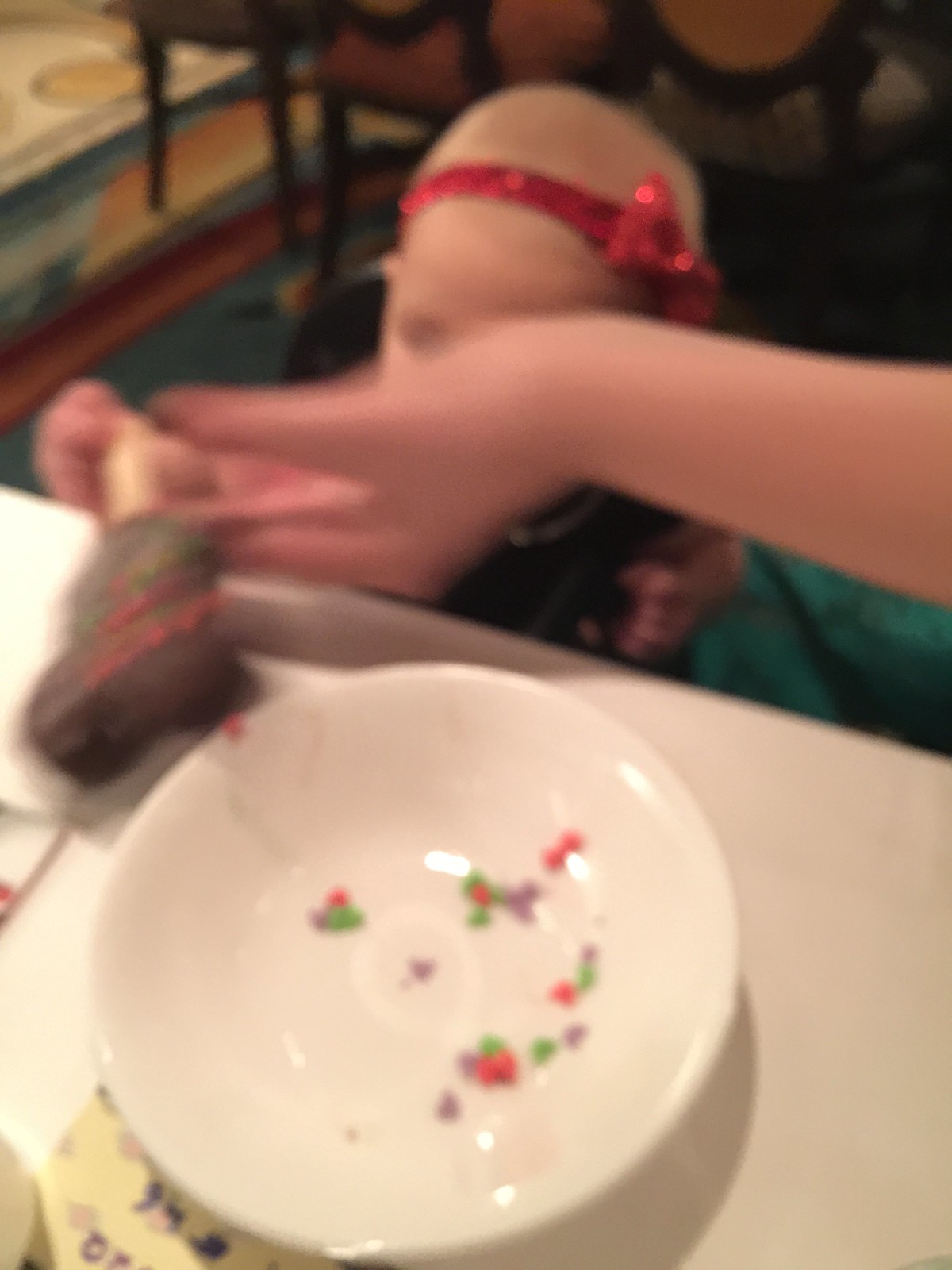In a somewhat blurry photo, a young baby—possibly not yet walking due to her small stature—is seen standing in the foreground. She has minimal blond tufts of hair and wears a bright red headband adorned with a bow. The baby's face is obscured by an adult's outstretched arm and hand, likely attempting to intercept her small right hand, which is reaching up towards a brown item on a stick, possibly a popsicle. In front of the baby, there's a table covered with a cloth that appears white but has a pink hue in the photo. On the table, a white bowl containing a sprinkling of colorful items, resembling red, purple, and green sprinkles, is visible. Behind the baby, the scene includes a vividly bright turquoise rug and a few wooden chairs.